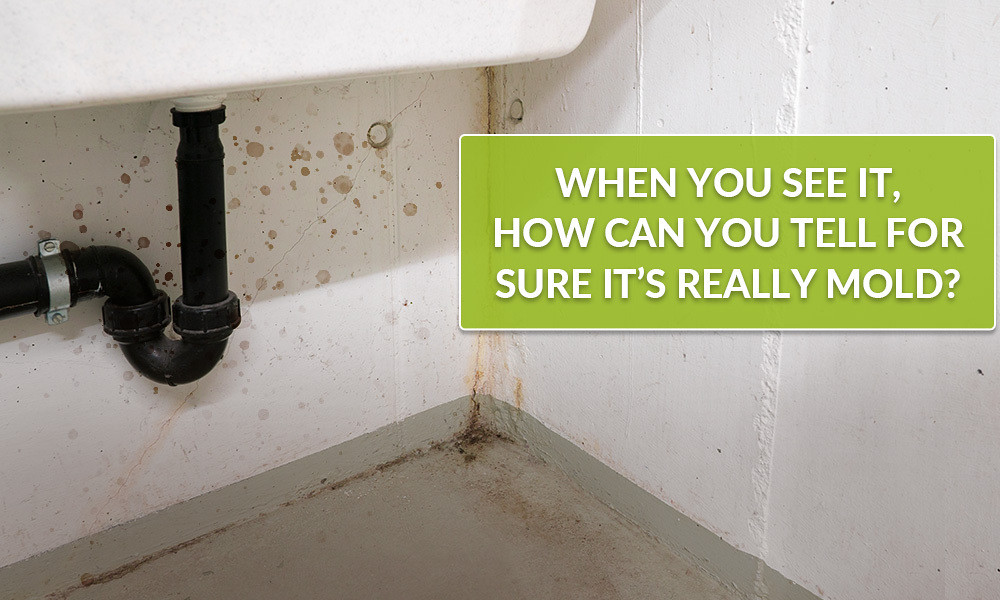This photograph, likely from an educational advertisement about mold identification, captures the area under a sink, featuring a prominent green rectangle with the text, "When you see it, how can you tell for sure it's really mold?" in white font. The focus is on a white wall marred by brown spots and possible mold, as well as a black PVC pipe. The piping loops downwards and is secured to the wall with a silver clamp. To the far right, there's a white tank connected to the plumbing. The bottom portion of the wall and the floor are painted gray, while the corner of the wall exhibits a noticeable crack with rust buildup and brown grime. This setup highlights the challenge in discerning mold presence based solely on visual inspection. The entire scene is depicted in shades of white, black, gray, green, and brown.